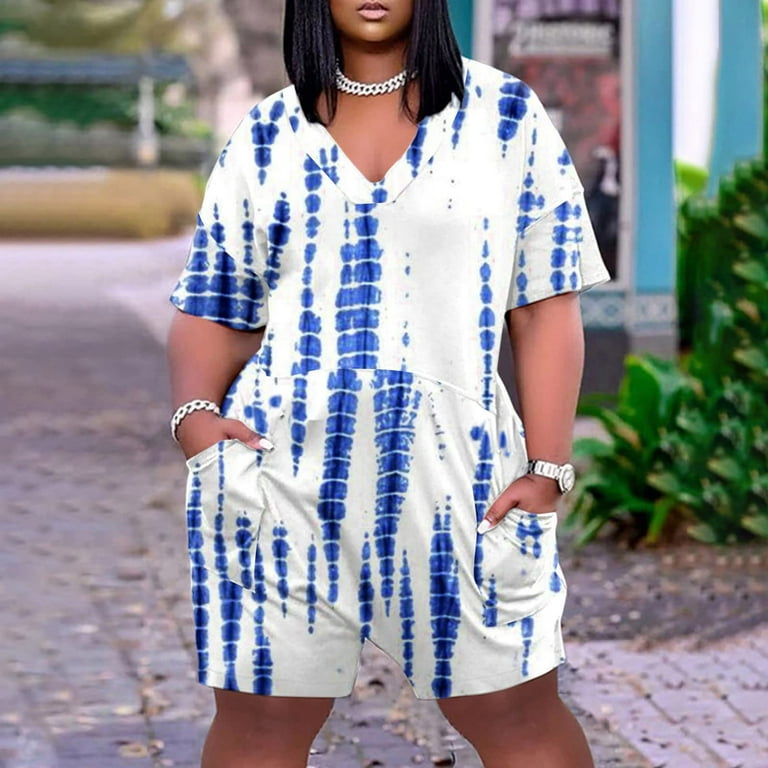The image depicts an African-American woman modeling a casual, white shorts jumpsuit adorned with navy blue tie-dye patterns forming vertical stripes and splotches. Her straight black hair falls to her shoulders, and she wears pink lipstick. Around her neck is a thick silver chain necklace, which matches the silver bracelet on her right wrist and the silver watch on her left wrist. Her hands are in the pockets of her jumpsuit, with her thumbs resting outside. Notably, her nails are painted white. The photograph shows her posing outdoors on a brick pathway, surrounded by tropical vegetation, including a green bush. In the blurry background, an aqua-colored building with a pinkish-reddish door and some additional structures in blue interspersed with red hues are visible. The image captures her from knee height up to just above her top lip, excluding her eyes from the frame, and conveys a warm, tropical setting.